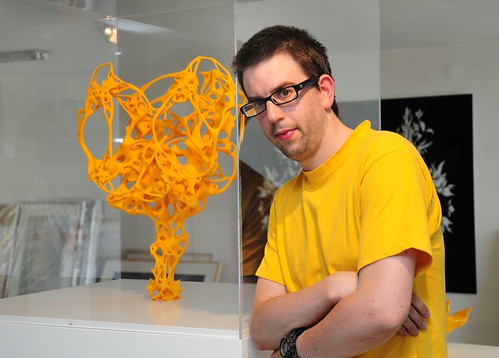This photograph captures a Caucasian man standing in an art studio, looking directly into the camera with his arms confidently crossed. He wears a bright yellow short-sleeved t-shirt, black-rimmed rectangular glasses, and a thick black wristwatch on his left wrist. His short, dark brown hair complements his stubbly beard and mustache. Positioned to the right side of the image, the man stands next to a display case on a white pedestal. Encased in glass, the case houses an abstract yellow sculpture composed of intricate, lace-like lines, resembling Swiss cheese in texture and form. The background features a black painting with white shapes partially obscured by the man's body. Additionally, several picture frames are visible, leaning against the left wall, adding to the studio's creative ambiance.